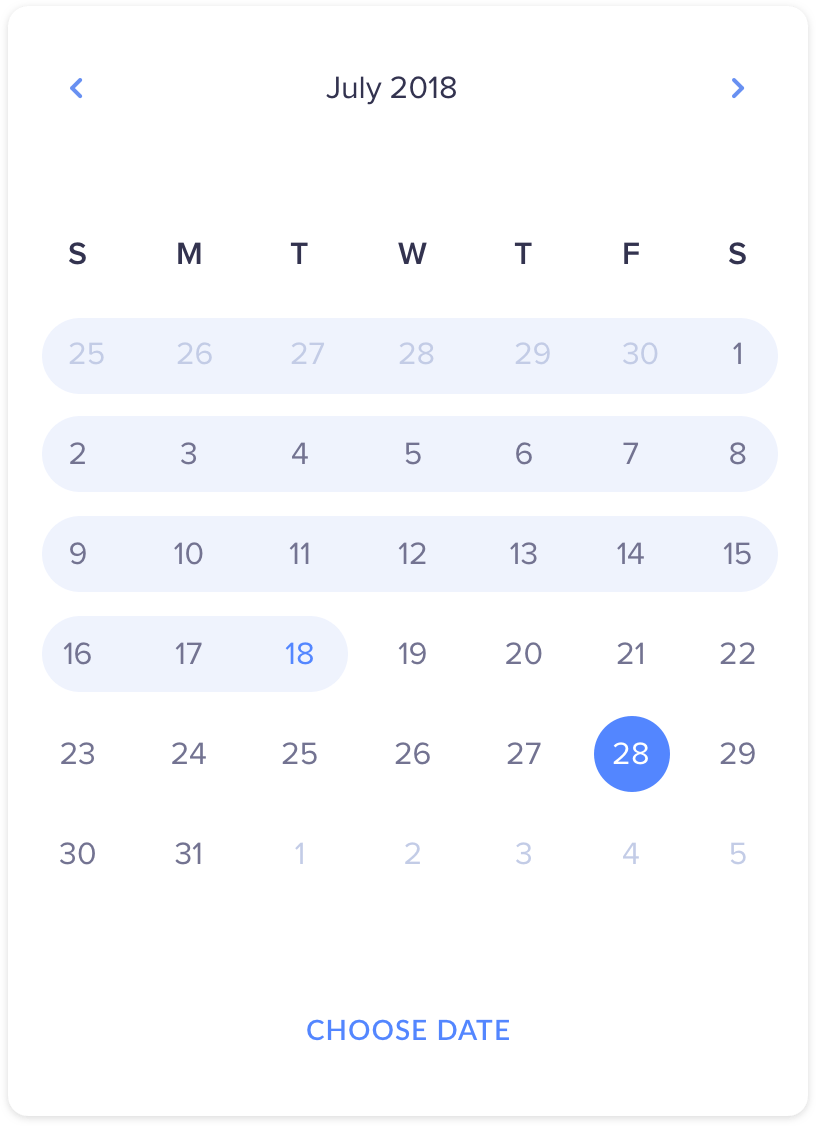This screenshot depicts a simple, minimalist calendar application interface. The background is white, providing a clean and uncluttered look. At the top, the heading "July 2018" is displayed in black font, centered between two blue arrows – the left arrow in the upper left corner and the right arrow in the upper right corner, allowing for navigation between months.

Directly below the month and year, the days of the week are labeled in black text: "SMTWTFS" (Sunday through Saturday). 

The calendar grid starts with the dates 25, 26, 27, 28, 29, 30, and 1, each enclosed within a light blue oval. These are followed by a second row of dates: 2, 3, 4, 5, 6, 7, and 8, also highlighted in light blue ovals. 

Subsequent rows continue this pattern with dates 9 through 15, and 16 through 18 all highlighted in the same manner. Below these, the dates continue without the light blue highlighting: 19, 20, 21, and 22, followed by 23, 24, 25, 26, and 27. The date 28 stands out with a solid blue circle around it and is displayed in white text, distinguishing it from the rest.

Moving on, the calendar displays dates 29, 30, and 31, followed by the first few days of the subsequent month, ending with dates 1 through 5.

At the bottom of the screenshot, the phrase "Choose Date" is prominently displayed in blue font, likely indicating a selectable action or prompt for the user.